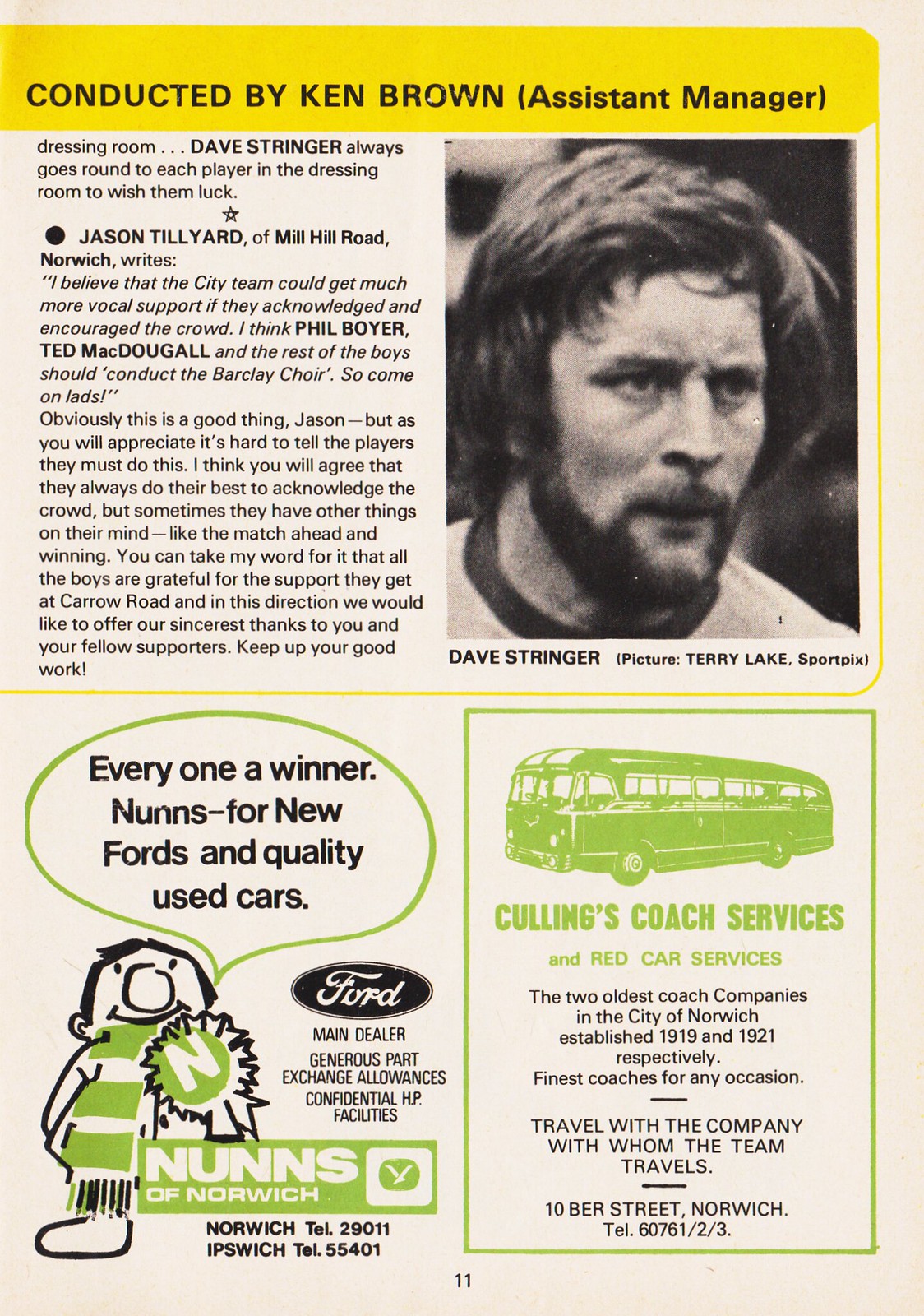This image depicts page 11 from an old sports magazine or soccer game program. The page is filled with various elements and detailed content, framed by a nostalgic aesthetic typical of vintage publications.

Across the top of the page, a yellow bar carries the header, "Conducted by Ken Brown (Assistant Manager)." This indicates a segment perhaps guided or written by Ken Brown. Below this header, the page continues mid-article in the top left column, suggesting a continuation from the previous page.

Prominently, the top right section features a photograph of a shaggy-haired man sporting a light beard, identified in the caption as "Dave Stringer pictured by Terry Lake Sport Picks." In the main text, it mentions how Dave Stringer makes a point to wish each player good luck in the dressing room.

The page includes interactive reader content, exemplified by Jason Tilliard of Mill Hill Road, Norwich, voicing his opinion on how the city's soccer team could benefit from encouraging vocal support among the fans. He mentions players like Phil Boyer and Ted McDougall, urging them to engage with the crowd and lead the Barclay Choir.

At the bottom of the page, advertisements cover the left and right corners. On the bottom left, there’s an ad for a Ford dealership, reading, "Everyone a winner, Nun’s for new Fords and quality used cars," accompanied by an illustration of a person with a green-and-white striped scarf holding a green ribbon. Below this, the logo reads "Nun’s of Norwich."

To the right, a second ad features a green-printed bus and promotes Collings Coach Services and Red Car Services. The ad emphasizes the companies' long-standing heritage, "The two oldest coach companies in the city of Norwich established 1919 and 1921 respectively," and boasts, "Finest coaches for any occasion. Travel with the company with whom the team travels."

The colors throughout the page include tan, yellow, black, light green, and gray, contributing to the vintage feel. Each element is meticulously placed, ensuring the page is informative and engaging for the reader. The page number 11 is centered at the bottom, ensuring readers can navigate through the publication seamlessly.